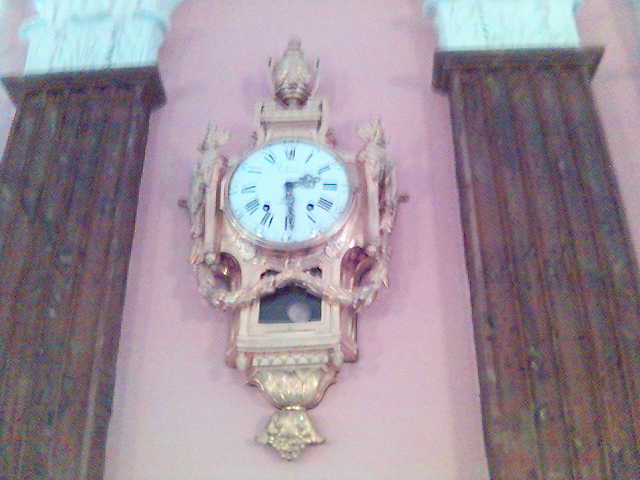This image showcases an antique clock with a distinctive goldish-pinkish hue. The clock features a tall and slender design, adorned with a clear glass window at the bottom that reveals a swinging pendulum. Below the pendulum, an intricate metal ribbon decorates the front and extends around the sides, adding to the clock's vintage charm.

The top portion of the clock is highlighted by an ornate, chalice-like decoration, creating an elegant focal point. The clock itself is flanked by two decorative pillars, painted in a rustic palette of browns and greens. Resting atop these pillars are statues that enhance the overall grandeur of the piece. The backdrop for this elegant clock is a wall painted in a soft pinkish color, complementing the antique aesthetic.